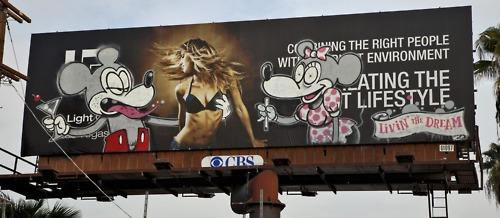The image portrays a billboard set against a clear daytime sky, with palm fronds visible on the right-hand side, suggesting an outdoor, tropical setting. The billboard itself, mounted on a brown base, features an advertisement of a blonde woman dressed in black bra and panties, her hair flying around her. The advertisement text includes fragmented phrases like "light," "the right people with," and "environment," alongside a visible "CBS" logo at the bottom.

Overlaying the original advertisement is vibrant graffiti art featuring exaggerated renditions of Mickey and Minnie Mouse. On the left side of the billboard, an intoxicated Mickey Mouse, depicted with half-closed eyes, a protruding red tongue, and no shirt, clutches a martini glass with an olive in his left hand while his right arm wraps around the waist of the woman in the ad. Mickey is drawn in gray with a white facial area.

To the right of the woman stands a graffitied Minnie Mouse, adorned with a pink bow and wearing a pink polka dot dress. Minnie is also depicted with an exaggeratedly long head and appears to be holding something in her right hand, although it is indistinct. At the bottom right of the billboard, meshing into the graffiti scene, is a white banner that reads "Living the Dream," harmonizing with the color scheme of the Minnie Mouse art. This bold street art transforms the commercial billboard into a striking, controversial piece reflecting a warped take on familiar Disney characters.